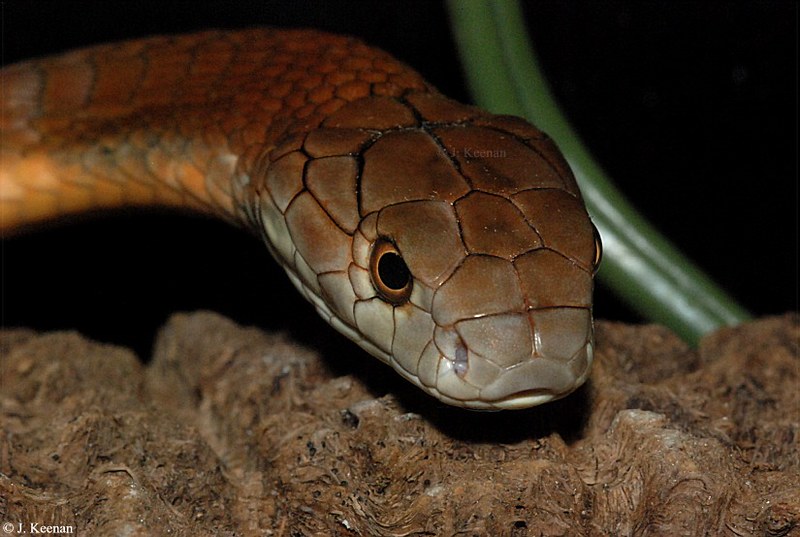The photograph is a close-up shot of a snake, predominantly capturing its head and about two inches of its body. The snake's scales feature a striking gradient of dark orange on top, transitioning to a lighter orange near the bottom, with its head showcasing a brownish hue. The defined scales give it a metallic, coppery appearance, especially around its neck. The snake's right eye, prominent in the frame, has a large cornea with a noticeable brown iris, while the left eye is barely visible at the image's edge. The mouth is almost closed, bordered by lighter-colored scales, possibly white. The background sets a dramatic contrast with the snake’s vivid colors; it is mostly dark, resembling nighttime, enhancing the snake's fierce, well-defined look. Alongside the snake is a green loop, likely a plant stem, and the lower part of the image reveals a brown, rock-like or sandy surface, suggesting natural terrain. Additionally, there is a green object, possibly a hose or plant stem, contributing to the scene's texture. The photograph is exquisitely detailed, capturing the snake’s intricate facial features, including its nostrils, making it appear almost lifelike.